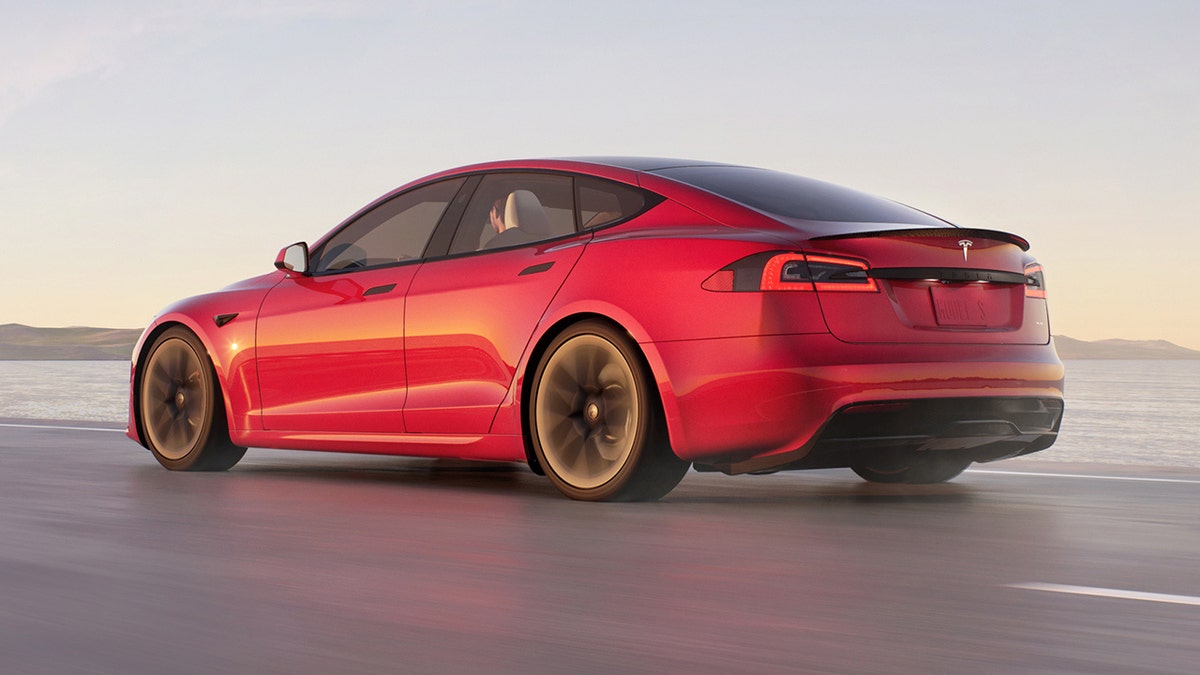In the image, we see a red Tesla sedan from a side and slightly rear perspective. The vehicle's tires, which are moving, suggest it is traveling on a gray road, marked by a single white line on the right-hand side. The car’s wheels are black with gray rims. The rear end of the Tesla, featured prominently to the right, has a black bumper and is adorned with a silver Tesla logo. The left side of the car is also red, complementing its sleek design. The windows are not tinted, revealing a glimpse of the gray interior and a partial view of a head in the driver's seat. The background is scenic, showcasing a blue body of water beneath a light blue sky, enhancing the serene setting of the scene.